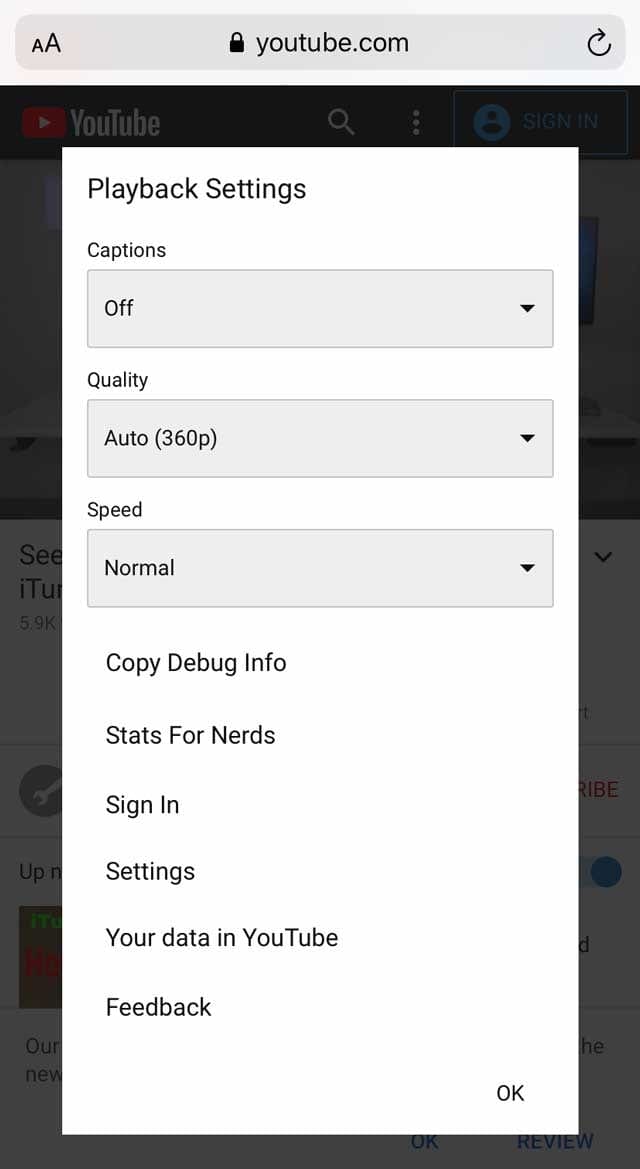This screenshot captures a YouTube video page viewed on a mobile browser, as indicated by the "YouTube.com" URL displayed at the top. The main screen of the YouTube page is grayed out, while a prominent white dialogue box titled "Playback Settings" overlays it. Within the dialogue box, three drop-down menus are visible; the first one, labeled "Captions," is set to "Off." The second drop-down menu is labeled "Quality" and is set to "Auto 360p." The third drop-down menu, labeled "Speed," is set to "Normal." Each drop-down menu is highlighted in a light gray rectangle with a small, downward-facing black triangle on its right side, indicating the menu can be expanded for more options. Below these settings, additional options are listed: "Copy Debug Info," "Stats for Nerds," "Sign In," "Settings," "Your Data in YouTube," and "Feedback." In the lower right-hand corner of the dialogue box, the option to confirm settings is marked with the letters "OK."